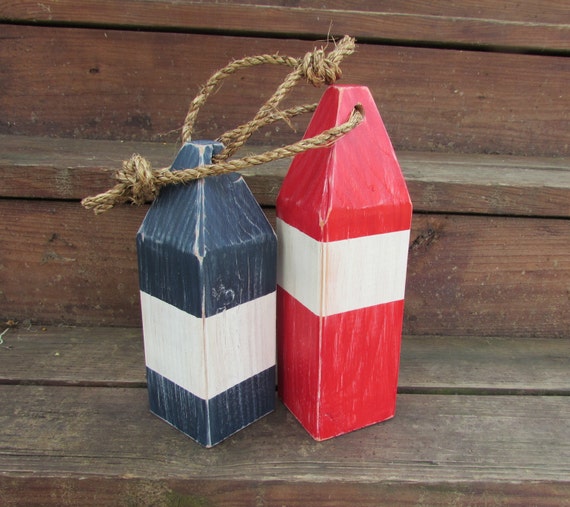The image captures a DIY marketing photo taken outside on light brown wooden steps featuring two decorative buoys that resemble brand-new crayons. Both buoys taper upwards to a pointed top with the wider base at the bottom. Each buoy has a white stripe near the top before angling inward, reminiscent of a four-way roof. The larger buoy is red with a wide white stripe positioned slightly higher, while the smaller buoy is blue with a similar white stripe positioned lower. Twisted brown ropes are tied around the tops, forming nautical-style knots, giving a sense of decorative maritime charm. The scene seems to include at least three steps, with the second and third steps displaying darker wood and visible slots. The two buoys are positioned closely together, their ropes dramatically overlapping across each other on the steps.